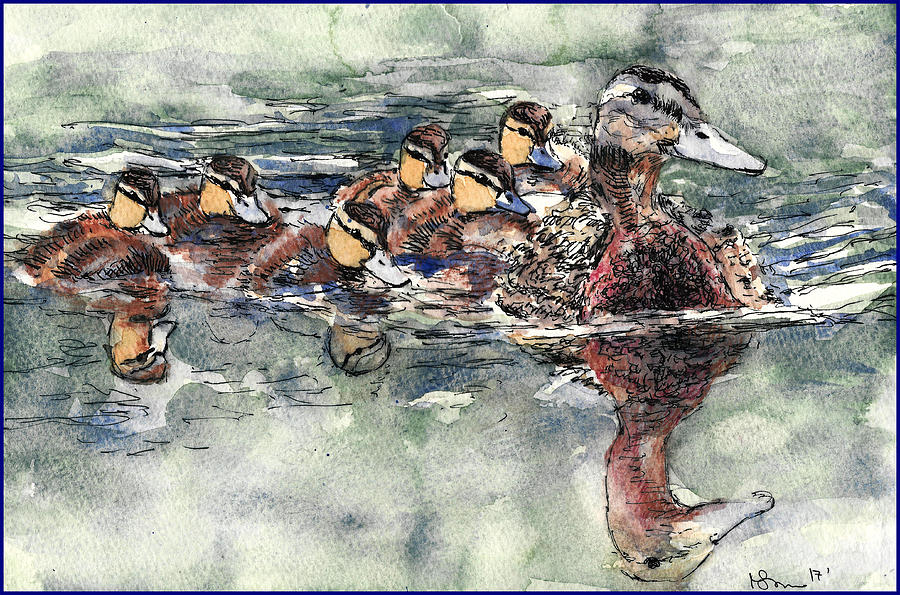This image is a delicately crafted watercolor painting depicting a serene family of ducks gliding through a calm stream. The centerpiece is a mother duck, distinguished by her reddish-brown body, with a yellow head and blue beak, leading a procession of six baby ducks, each with orangish-brown feathers and yellow heads. The soft pastel hues in shades of blue-gray beautifully blend to illustrate the gentle ripples and reflections in the water. The tranquil scene captures the baby ducks closely following their mother, with their mirrored reflections subtly distorted by the light movements in the water, giving a sense of gentle tidal waves. Elegantly painted, the artwork exudes a somber, yet peaceful atmosphere, enhanced by the artist's signature in the bottom right-hand corner.